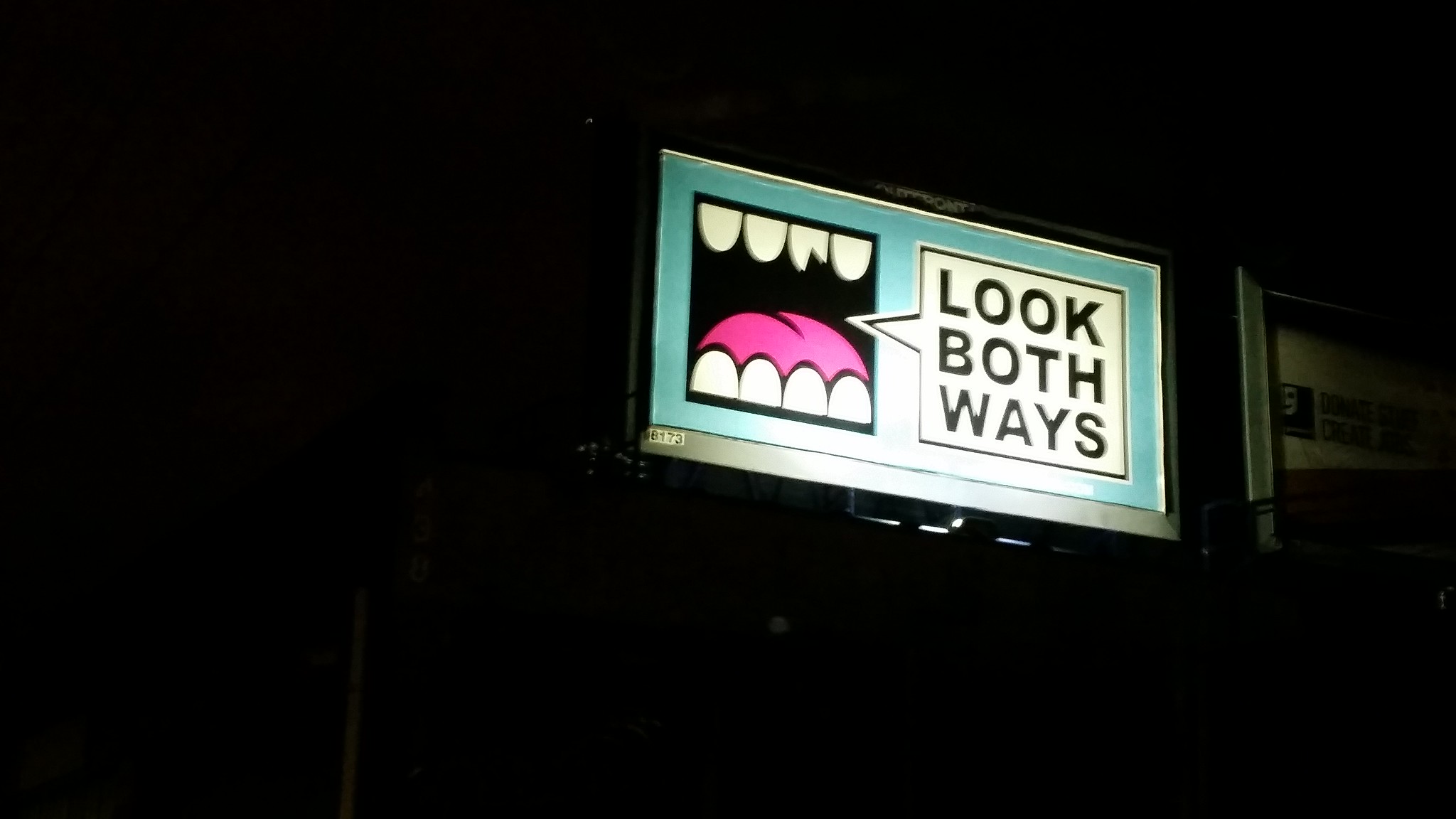A nighttime photograph captures an illuminated billboard set against a pitch-black sky. The billboard is turquoise and rectangular. On the left side of the sign, there's a square-shaped mouth with rounded teeth and a bright white tongue at its center. Emanating from the mouth is a speech bubble with the message "LOOK BOTH WAYS." The text is in bold black, all capital letters on a white background, emphasizing the importance of the message. Adjacent to this main billboard, there appears another sign, likely for Goodwill, identified by a partially visible logo consisting of blue and a white smiling face. This secondary billboard is muted and in shadow, making its details mostly unreadable, but it appears to be light in color, possibly white.